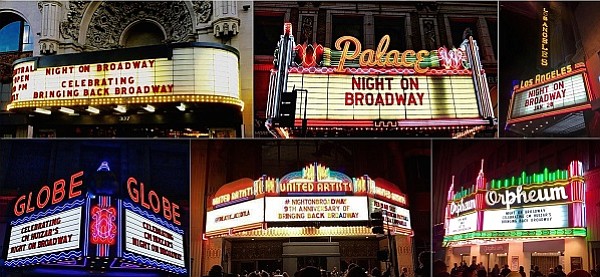The photograph is a collage of six different movie theater matinee boards, each showcasing an event titled "Night on Broadway." The composition features three images on the top row and three on the bottom. Starting from the top left, the first image is an ornate stone building with a white matinee board displaying in red text: "Night on Broadway, Celebrating Bringing Back Broadway." The second photograph in the center features a similarly styled white matinee board with red text that reads "Night on Broadway," accompanied by a neon sign above it with red letters outlined in yellow that spell "Palace." The top right image shows a board under the vertical marquee letters "Los Angeles," with the horizontal board beneath it also reading "Night on Broadway."

On the bottom row, the first image shows a theater with a sign that reads "Globe," and features small, unreadable text below it. The center photograph shows a sign that has three smaller signs on either side, but the text is also too small to be legible. Finally, the bottom right picture displays a theater with the name "Orpheum" at the top, and some unreadable text below. All six theaters share the common theme of promoting the event "Night on Broadway," with most utilizing red text on white boards, and several incorporating additional colored neon signs and ornate architectural details.